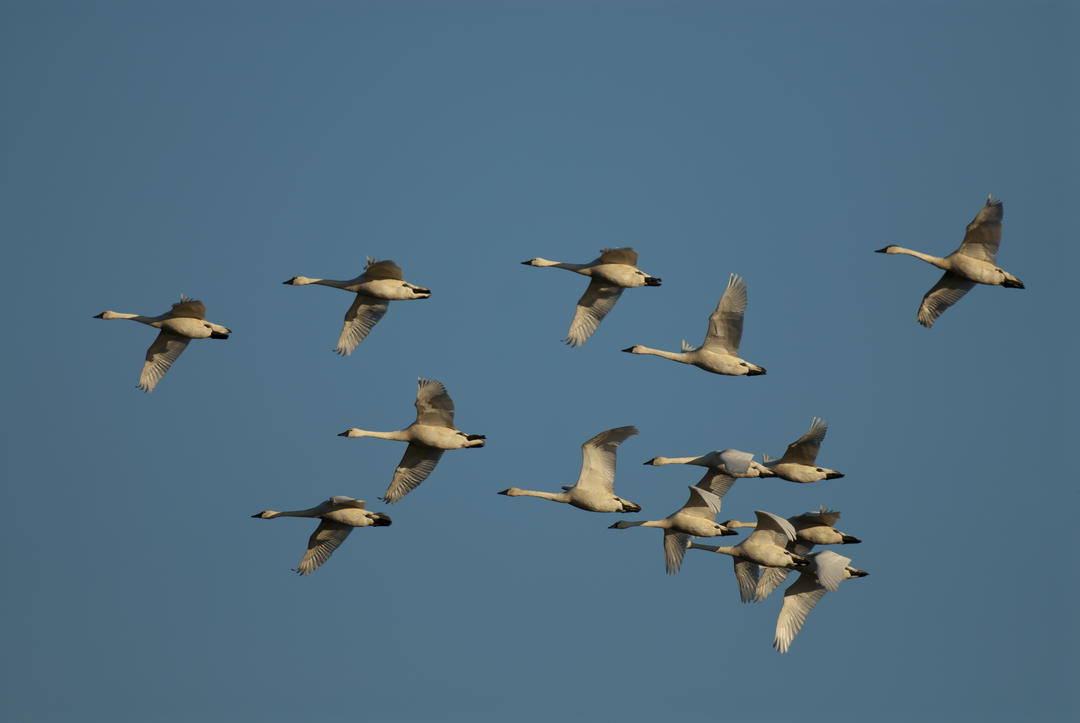This vivid, color landscape photograph captures a flock of Canadian geese soaring through a bright, clear blue sky. The image, taken from a high vantage point, presents a close-up view of the geese in mid-flight, highlighting their creamy white underbellies, darker gray wings, and distinctive black heads with long, white necks. The geese are seen flying toward the left side of the image, with a group of five forming a perfect V in the center and trailing behind them, nine more geese that appear to be attempting to get into formation. The natural daylight accentuates the crispness and clarity of the photograph, emphasizing the details of the geese's spread wings against the vivid sky. The overall composition showcases the grace and organization of the flock, representing realism in photographic art.